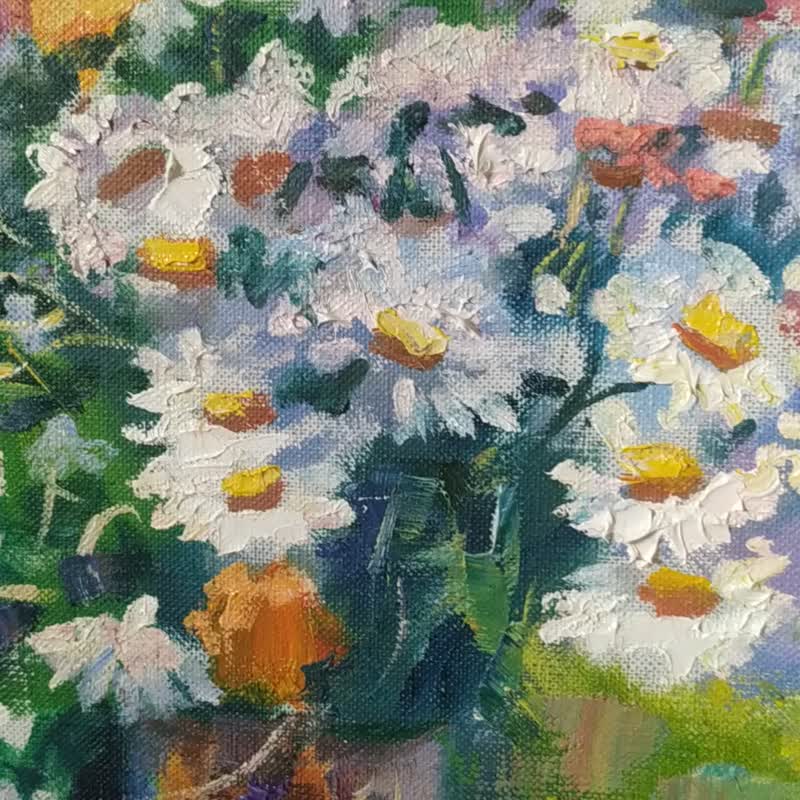The image is an oil painting featuring a striking bouquet of flowers, predominantly white daisies with yellow-brown centers. The composition includes a range of around 10 to 15 white daisies adorned with green leaves on stems that blend into grassy, varied green hues—from light to dark—with touches of blue and white. The painting is characterized by thick, textured paint application, particularly around the petals, which lends a smudged, yet gentle appearance as though the flowers were dipped in paint and carefully laid down. Adding complexity, there are orange and black flowers interspersed among the daisies, with some displaying red and black centers. The arrangement fades gracefully towards the bottom into earthy browns and tans. Additionally, sporadic bursts of red and black add visual interest, and the background foliage is lush and abundant, incorporating vibrant green leaves throughout. Overall, the painting conveys a sense of a densely packed, colorful floral scene that is both beautiful and somewhat chaotic, making it challenging to distinguish individual flowers within the jumbled array.